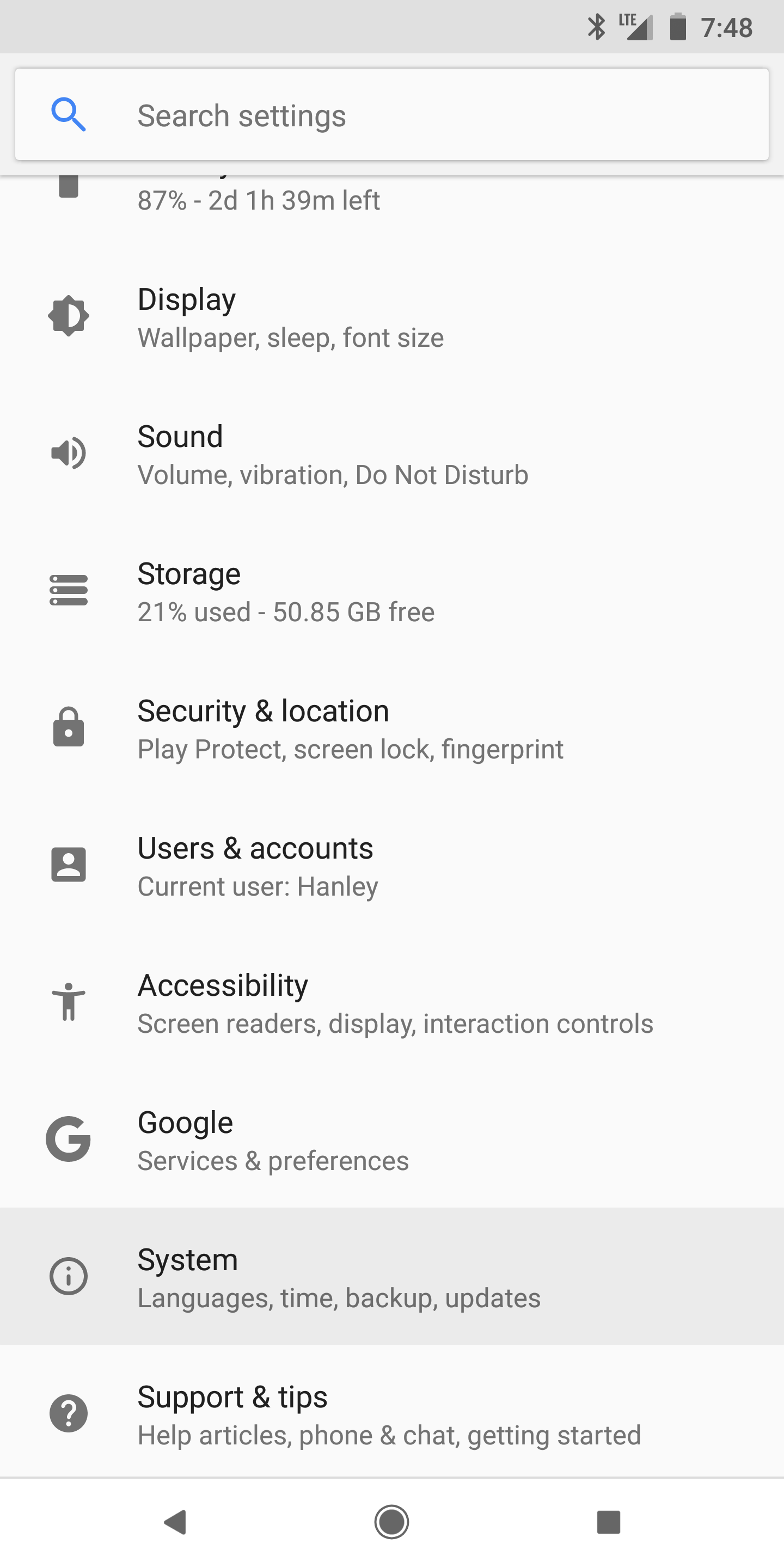The image depicts a smartphone screen with a detailed interface. At the top, there's a slim grey panel displaying various status icons on the right: a Bluetooth icon, signal strength indicator, a nearly full battery indicator, and the clock showing 7:48. Below this panel is a search field for entering search criteria.

Further down, there is a list of settings, each accompanied by an icon on the left, a title, and a brief explanatory text:
1. The first entry shows "87%", but the icon is unclear.
2. "Display" settings include options for wallpaper, sleep mode, and font size.
3. "Sound" settings offer adjustments for volume, vibration, and Do Not Disturb mode.
4. "Storage" is listed as 21% used, with 15.85 gigabytes free out of the total capacity.
5. "Security & Location" settings allow for configuration of Play Protect, screen lock, and fingerprint options.
6. "Users & Accounts" indicate the current user as "Hanley."
7. "Accessibility" features include screen readers and display/interaction controls.
8. "Google" settings manage services and preferences related to Google.
9. "System" settings provide configuration for languages, time, backups, and updates; this section is currently selected.
10. "Support & Tips" offers help articles, phone and chat support, and getting started guides.

The user interface is designed to be intuitive, presenting a comprehensive overview of the smartphone’s settings and options.